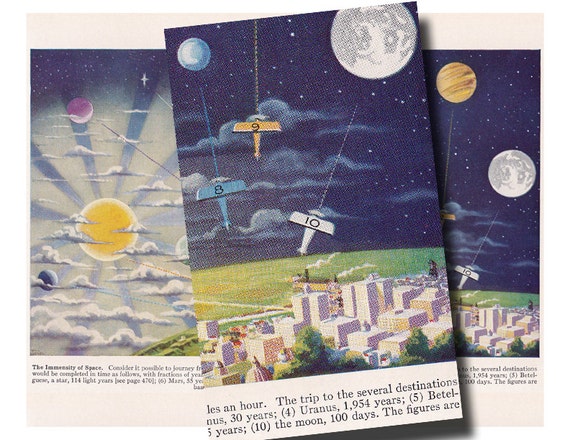The image depicts a detailed arrangement of space-themed illustrations and text spread across three separate pages or pamphlets, presented in a layered fashion. In the background, two pages are partially visible, while a foreground page is prominently displayed. This foreground image shows a striking depiction of a blue sky filled with stars, a moon, another celestial body (potentially Uranus), and a sprawling metropolitan area with green fields below. The text at the bottom of these pages mentions various travel durations to different space destinations, although some of it is cut off, listing these intervals: “less than an hour,” “30 years to number four, Uranus, 1,954 years,” and “100 days to the moon,” with a partially folded section that likely contains additional details.

The visible page or pamphlet above carries an illustration of three airplanes each marked with numbers—8, 9, and 10—seeming to launch towards the moon within a dark sky dotted with white clouds. Below these airplanes is a cityscape dominated by tall white buildings and skyscrapers, transitioning into a large grassy area. The imagery on what appears to be the inside of the card features a bright yellowish-orange sun with blue sun rays set against a sky interspersed with fluffy white clouds and a grassy hill underneath. The visual elements are predominantly in shades of blue, white, yellow, and tan, contributing to a cohesive color palette across the illustrations.

Moreover, both a section of text in black and a folded, poster-like quality of the material suggest that it might serve as an interactive or expansive visual display, with perforations or folds revealing more details when manipulated. The interplay of light and shadow from overlapping sections accentuates the dimensionality of the presentation, creating a sense of depth and layered narrative in the visual storytelling.